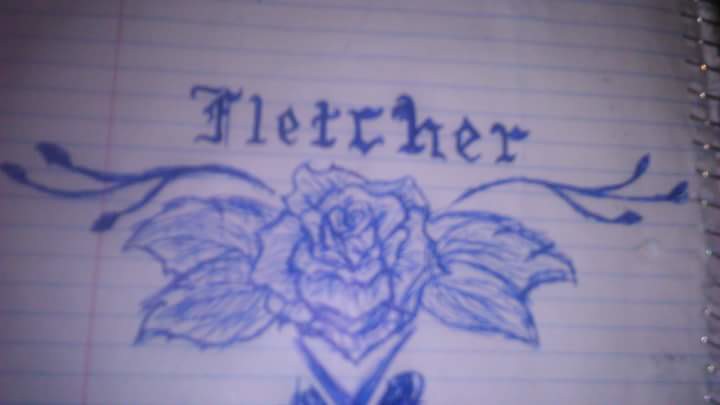The image showcases a notebook with white paper as the backdrop, featuring blue horizontal lines typical of ruled paper. On the right side, spiral rings are visible, indicating it is a spiral-bound notebook. Towards the left edge of the sheet, a bold red margin line can be seen. At the top of the page, the name "Fletcher" is stylishly written in an artistic font, with each letter clearly detailed as F-L-E-T-C-H-E-R. At the bottom of the page, a meticulously drawn rose is centered. The rose features intricately detailed petals that extend gracefully to both the left and right. The inner part of the rose is expertly shaded to give a blossomed, three-dimensional appearance using blue ink, evoking the style of a tattoo. The petals and leaves are carefully outlined and filled with shades of blue, adding depth and texture to the design.